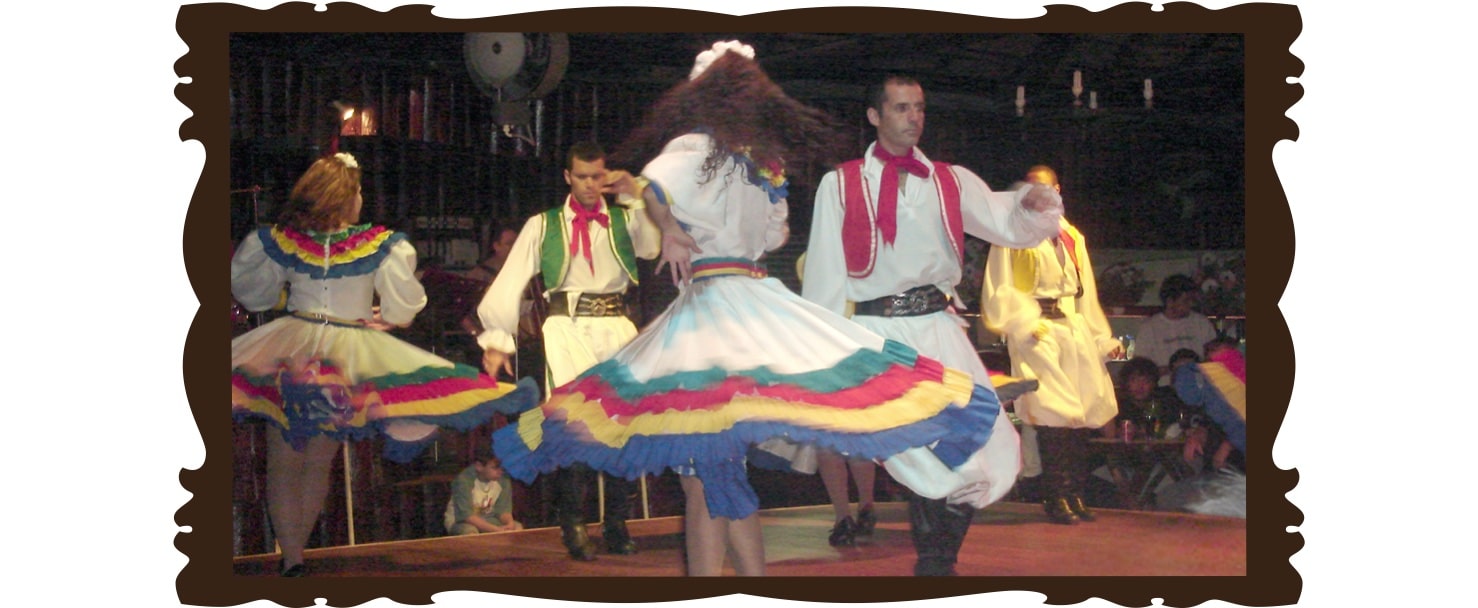The image features a lively cultural event showcasing six dancers, three men, and three women, who are engaged in a traditional dance. The setting appears to be a festive environment, possibly a party or a restaurant, evident by the visible tables and potential drinks and food in the background. The performers are likely of Mexican heritage, indicated by the traditional attire they are wearing.

The female dancers are dressed in elegant white dresses adorned with vibrant, multi-colored stripes at the bottom of the skirts, which include hues of green, red, yellow, and blue. These colorful accents are mirrored around the collars of their dresses. The women’s skirts flare out beautifully as they spin, creating a striking visual reminiscent of a colorful umbrella. Their dresses also feature puffy sleeves that add to the festive aesthetic.

The male dancers complement the women with their coordinated outfits. They wear white button-down tops and white pants tucked into black calf-high leather boots. Each man sports a red tie, and their outfits are accessorized with vests of different colors: one wears a red vest, another a green vest, and a third in the background appears to be wearing a yellow vest. The men also have black belts cinching their waists.

The image captures the energetic atmosphere of the dance, reflecting a rich cultural heritage through the performers' traditional clothing and spirited movement.